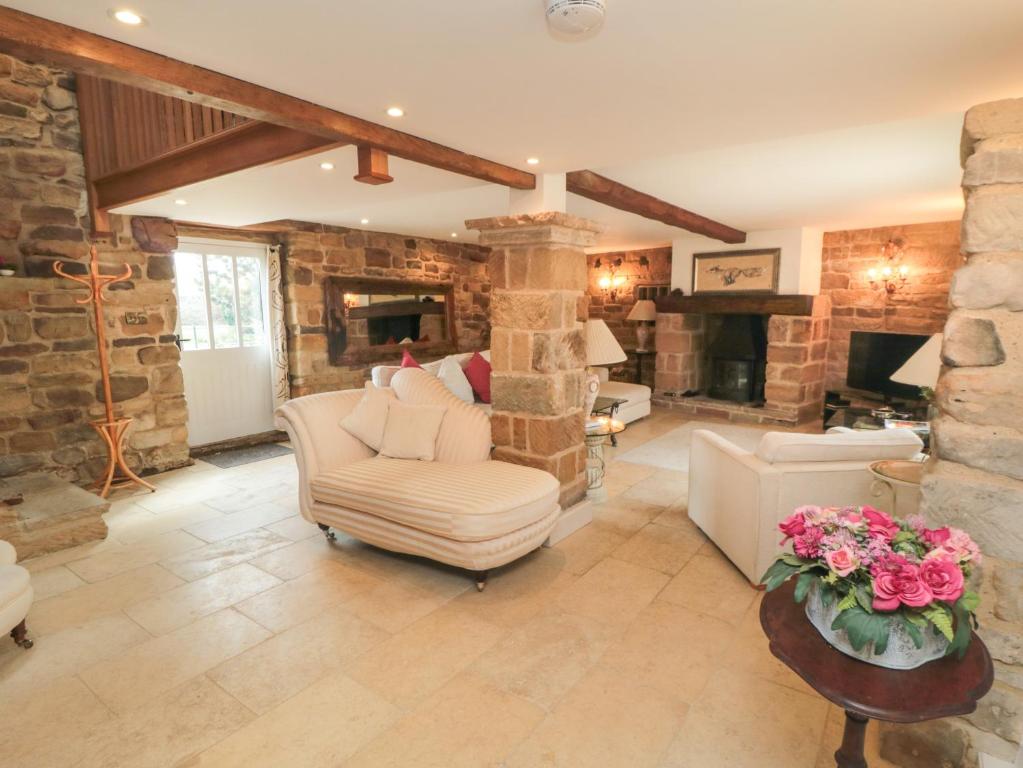This photograph showcases a spacious, rustic living room or den that resembles a lodge, featuring earthy, textured design elements. The large, open room has walls adorned with a mix of uneven, multi-colored bricks and stone accents in shades of brown and tan. The bleached white wooden floor contrasts with the robust stone and brick used throughout the space. The foreground presents a wooden table, round-topped, with a vibrant display of pink flowers, adding a touch of color amidst the earthy tones.

Central to the room is a rough stone or brick pillar that supports the ceiling. Surrounding this pillar are several pieces of cream-colored seating furniture, including white couches, chairs, and a chaise lounge, creating inviting conversation areas. Wooden beams stretch across the white ceiling, adding to the rustic aesthetic. There are multiple white lamps placed strategically around the room, contributing to the warm, cozy ambiance.

In the background, you can see a stately brick fireplace on the right side of the room, with a painting or picture hanging above it, and opposite, a mirror framed in wood. A white door with glass panes at the top lets in natural light and offers a view of the outdoors, further illuminated by bright light that pours in through the nearby windows. A wooden coat rack stands next to the door, enhancing the home's welcoming feel.